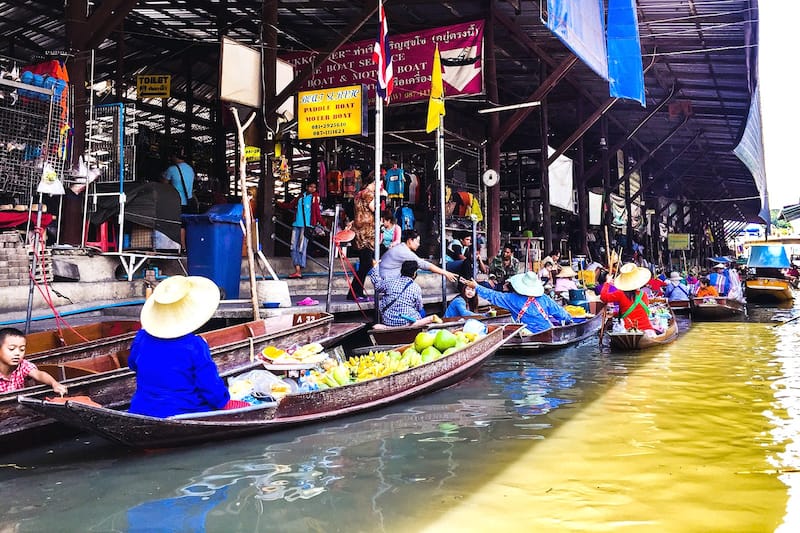The image depicts a bustling waterside market in Southeast Asia, potentially Thailand, characterized by an array of longboats resembling canoes, filled with various fruits and produce. Boatmen, predominantly women wearing wide-brimmed sun hats and dressed in dark blue, red, and yellow clothing, are conducting business with customers. On the left-hand side of the river is a covered marketplace area, teeming with activity under an awning supported by metal rafters. The water appears greenish and polluted. The market building extends right to the water's edge and features a variety of stands selling different items, including t-shirts. A boy is seen pointing at another boat, highlighting the lively and chaotic atmosphere. People on the boats are exchanging money and goods with those on land or from the edge of the market, emphasizing a vibrant and dynamic scene captured in daytime. The signage, mostly in English, and industrial equipment add to the complexity of this live, colorful photograph.